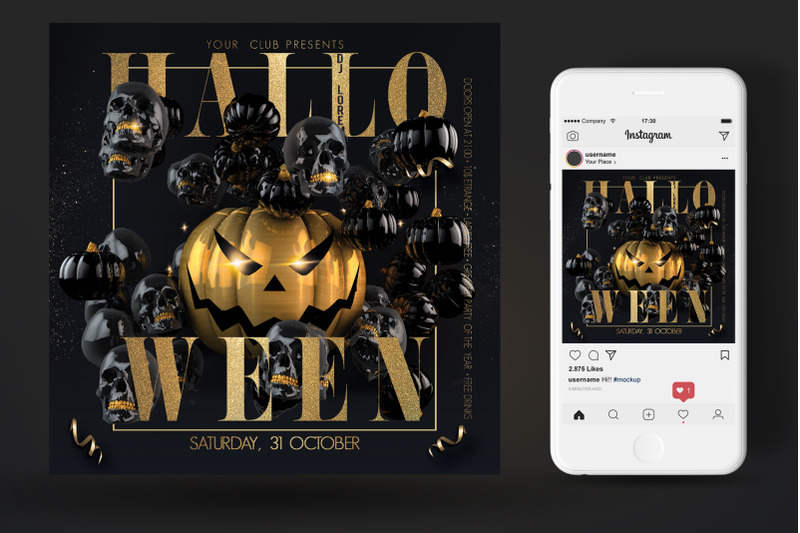This detailed image displays an intricate Halloween advertisement. The composition is divided into two main sections: on the left, a square poster resembling a napkin, and on the right, an iPhone displaying the poster within an Instagram feed.

The left section, the poster, prominently features the words "Halo" at the top and "Ween" at the bottom in elegant gold font. The background is intricately designed with an array of black and gray skulls and pumpkins, creating a spooky atmosphere. At the heart of the design, a large, menacing jack-o'-lantern with slanted, malevolent eyes, a triangular nose, and a jagged, open mouth stands out. This gold pumpkin adds a touch of eerie sophistication to the composition. Additional details include the date "Saturday, 31 October" inscribed at the bottom, flanked by gold ribbons in the lower left and right corners. The text "Your Club Presents" is small and at the top, while the letters "D-J-L-O-R-E" appear vertically within the second "L" of "Halo." The skulls, some grinning with gold teeth, add to the chilling theme.

On the right, the iPhone screen displays the same poster within an Instagram post layout. The image is replicating the square advertisement, showing the typical features of an Instagram feed. The interactive elements are visible, including the heart (for likes), speech bubble (for comments), and paper airplane (for sharing). The post has garnered 2,875 likes, and a comment from user "username75" mentions "#mockup." The profile image of the poster's uploader is an empty gray circle with a pink outline. At the bottom of the screen, the like option is active, accompanied by a pop-up with a red background, a white heart, and the numeral "1" in white, indicating engagement.

Overall, this image combines digital and traditional promotional elements to effectively advertise a Halloween event, utilizing a creative and visually engaging design.